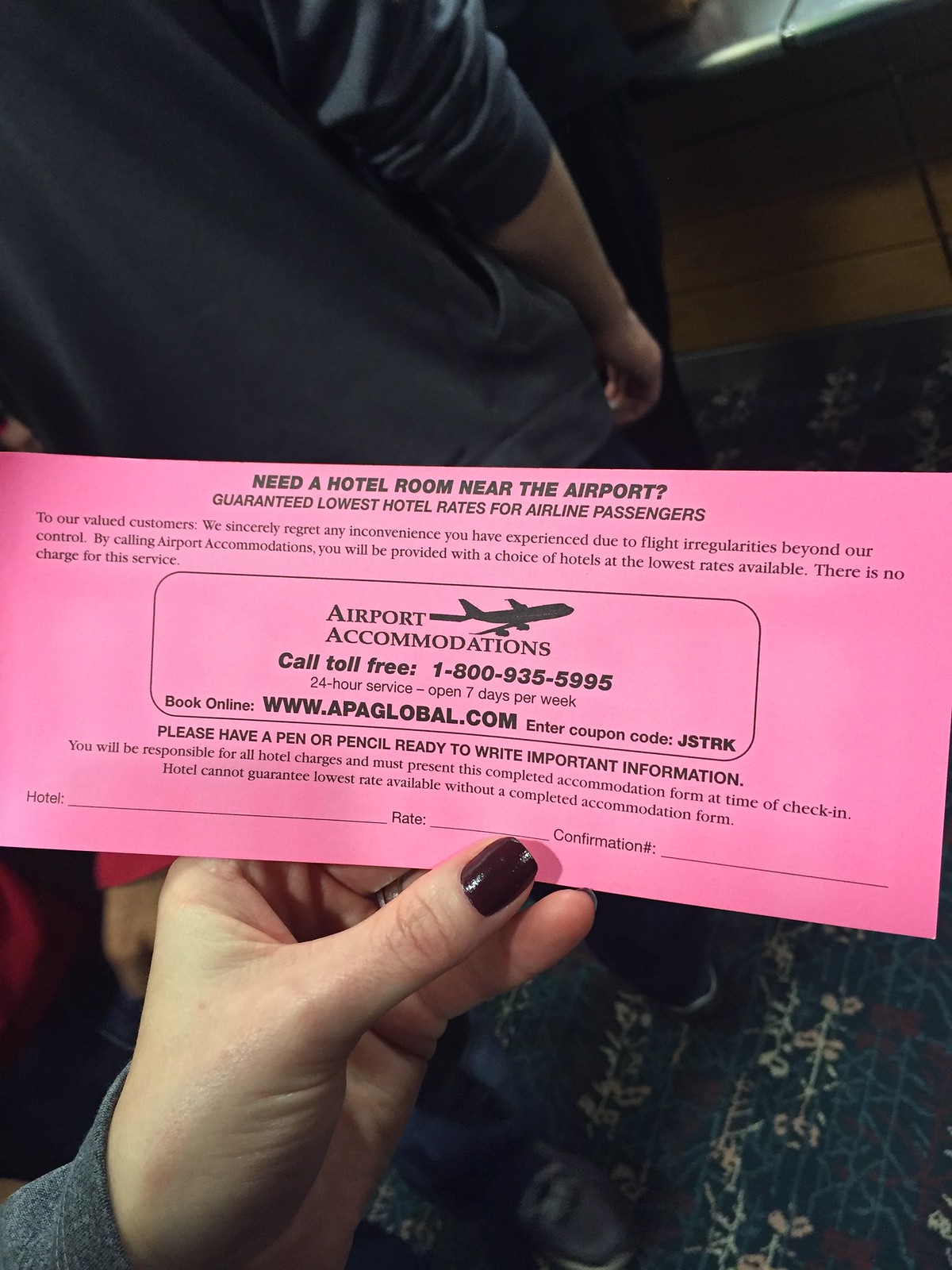In this photograph, a person—whose hand, sporting burgundy nail polish, emerges from the lower left corner—is holding a wide, pink ticket. The ticket displays black text that reads, "Need a hotel room near the airport? Guaranteed lowest hotel rates for airline passengers." Below this text, there's a section featuring an image of an airplane and the heading "Airport Accommodations" along with the toll-free number 1-800-935-5995. Additional tiny, difficult-to-read text follows, and instructions to "Please have a pen or pencil ready to write important information." The ticket also includes a website, www.apaglobal.com, and a coupon code, JSTRK. There are spaces designated for hotel rate and confirmation number. The person holding the ticket appears to be wearing a grey sweater and seems to be standing in line, as part of another person is visible in front of them, along with carpeted flooring and possibly the edge of a denim skirt.